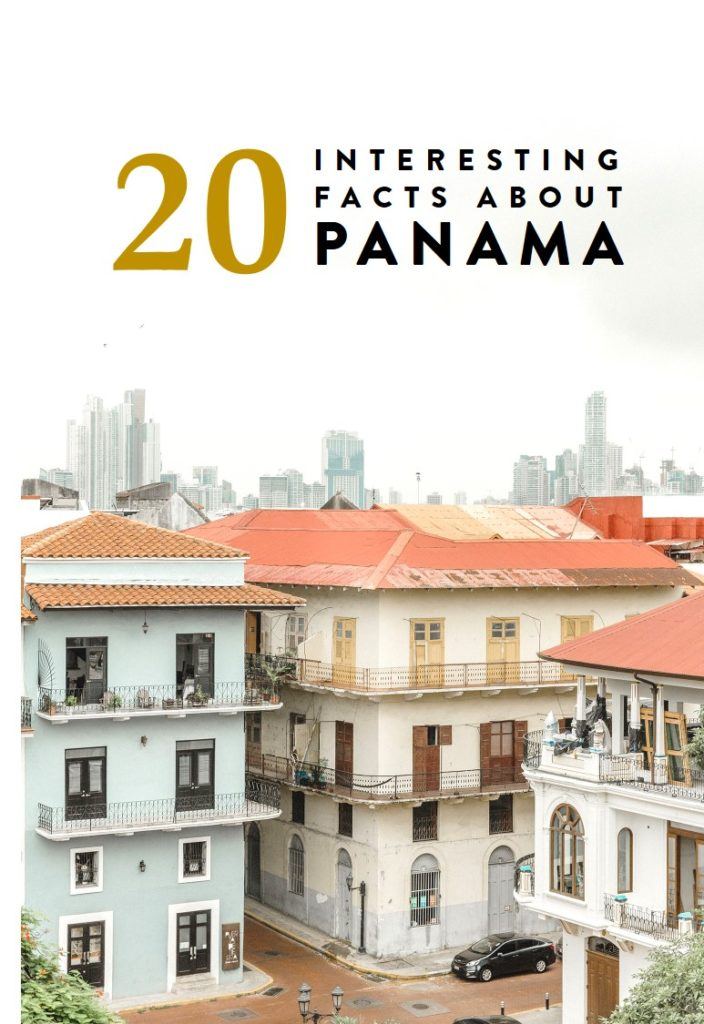This image presents an intricate, magazine-like cover that features detailed architectural scenes. At the very top, the number "20" is prominently displayed in dark gold, immediately drawing attention. Adjacent to this, in bold black text, are intriguing facts about Panama, inviting readers to delve into the content. 

The background showcases a white sky, setting a clean backdrop for the structures below. Dominating the center are tall buildings in various shades of gray and white, emphasizing urban contrast. To the left, a four-story building stands out with its charming terracotta roof. The façade is painted a delicate light blue and adorned with two black windows per floor. These windows open onto white balconies, secured by black railings, adding a touch of elegance.

On the right, a bright orange roof crowns a three-story building. Its exterior is a soft white or light beige, with a harmonious color scheme for the doors and windows. The top level features light brown doors, whereas the second level has dark brown accents, and the ground floor boasts cathedral-shaped windows, enhancing the visual appeal.

Below, the street is depicted in a sandstone hue, bringing warmth to the scene. A sleek black car is parked in front, adding a modern touch. Finally, the rightmost building mirrors the previous one’s orange roof. This edifice, painted in white, has its top level cluttered with what appears to be doors or building materials, hinting at ongoing construction or renovation.

Overall, the cover meticulously captures the vibrant and eclectic urban landscape, blending historical architecture with contemporary elements.